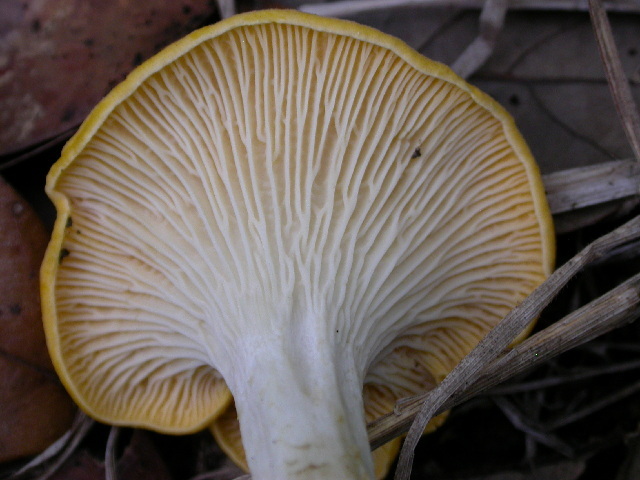This image is a close-up view of a large mushroom taken from underneath, looking up. The mushroom boasts a white stem and a cap that transitions from white on the underside to a light yellow on the top. The cap features a delicate, flowy texture reminiscent of flower petals, with pronounced white veins visible underneath. The setting appears to be a forest, as indicated by the presence of surrounding elements like brown and white tree branches and leaves, although these background details are somewhat blurry and dark compared to the sharply focused mushroom.